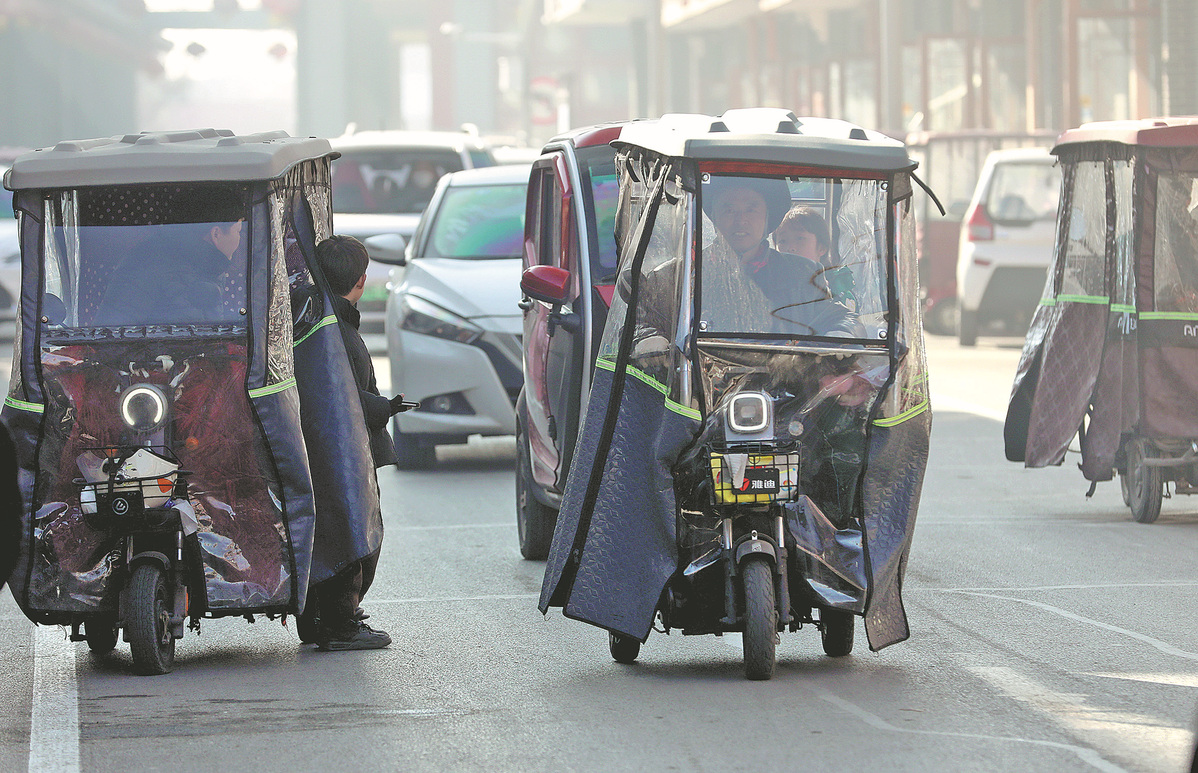The image depicts an outdoor, daytime scene in a bustling urban environment, likely in an Asian country. The main focus is a motorized tricycle, commonly referred to as a tuk-tuk. This small three-wheeled vehicle, which often serves as a taxi, features one wheel in the front and two in the back, complete with a basket and a headlight at the front. The tuk-tuk has a windshield and a roof supported by metal bars, and its sides are enclosed with plastic curtains that protect against the elements. The top part of the curtains is clear, while the bottom appears more durable, resembling a tarp. The driver, wearing a coat and a large hat, is visible through the windshield, though somewhat obscured by reflections. A passenger sits behind him in the enclosed rear section. The vehicle is on a paved road marked with white lines, in the midst of other traffic including modern sedans, SUVs, and hatchbacks. The background shows out-of-focus buildings, adding to the sense of a densely populated city. People are also visible near other tuk-tuks, presumably waiting for passengers.